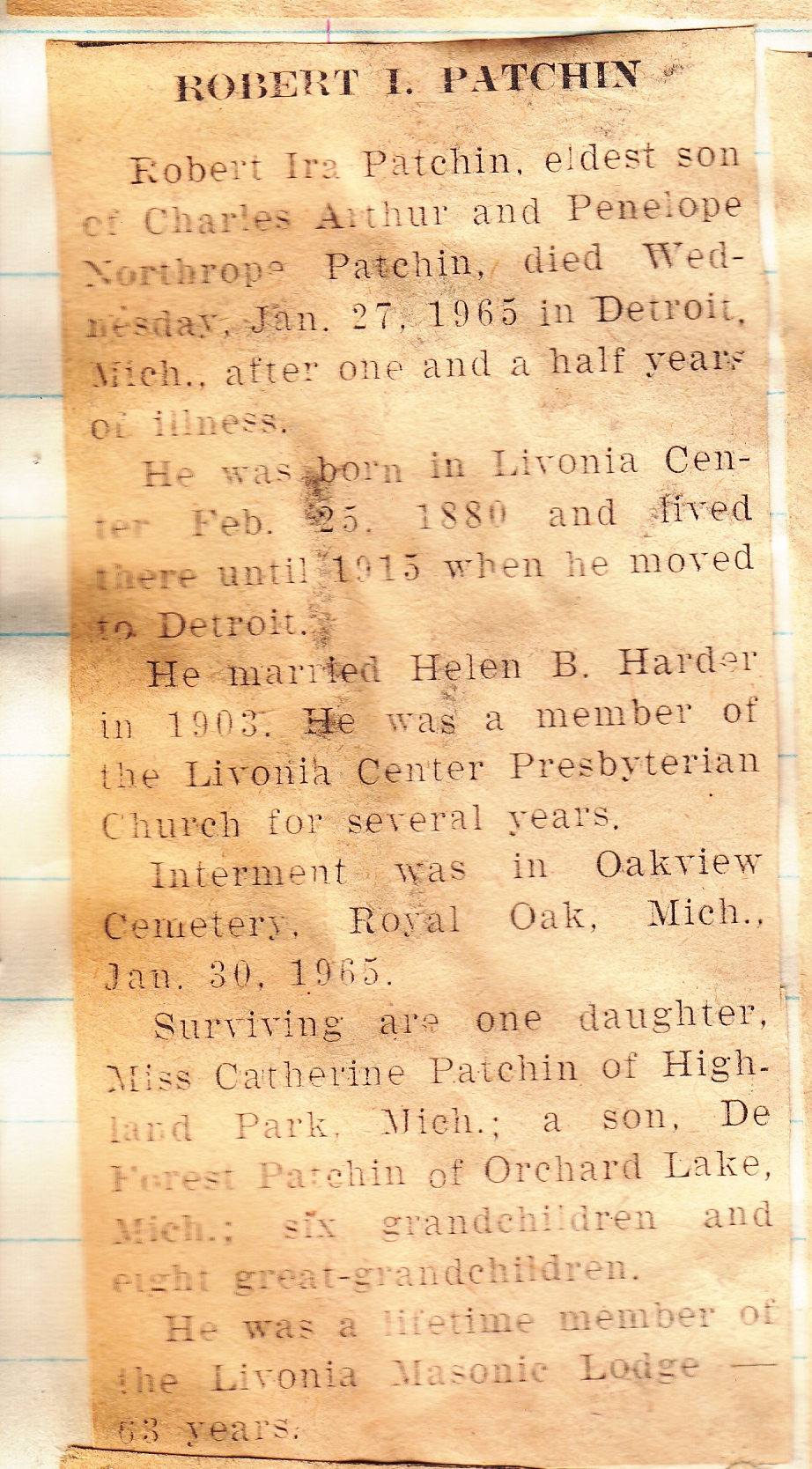This image features an aged and tan-stained newspaper clipping that serves as an obituary for Robert Ira Patchen. The clipping, showing clear signs of wear and deterioration, is attached to a sheet of ruled binder paper, with visible blue lines along the left edge. The headline reads "Robert I. Patchen" in bold, black letters.

According to the obituary, Robert Ira Patchen, the eldest son of Charles Arthur and Penelope Northrop Patchen, passed away on Wednesday, January 27, 1965, in Detroit, Michigan, following a one-and-a-half-year illness. Robert was born on February 25, 1880, in Livonia Center, and moved to Detroit in 1915. He married Helen B. Harder in 1903 and was affiliated with the Livonia Center Presbyterian Church for several years. His final resting place is the Ophie Cemetery in Royal Oak, Michigan, where he was interred on January 30, 1965. Robert is survived by his daughter, Miss Catherine Patchen of Highland Park, Michigan; his son, DeForest Patchen of Orchard Lake, Michigan; six grandchildren; and eight great-grandchildren. He was also a lifelong member of the Livonia Masonic Lodge, having been a member for 53 years.